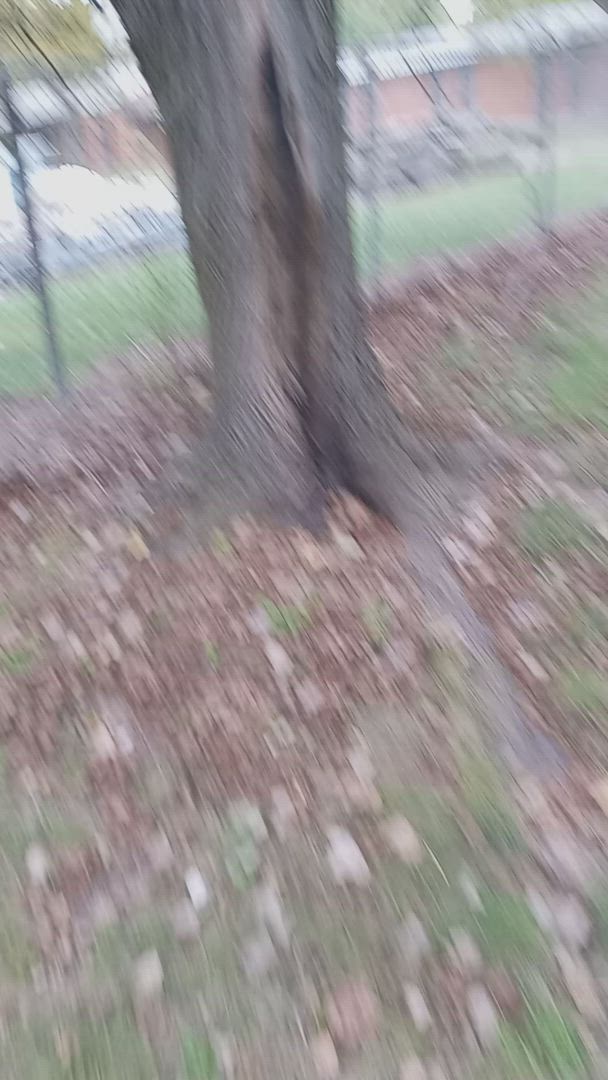This photograph appears to be taken outdoors and is notably out-of-focus. In the foreground, the ground is covered with a mix of green leaves and scattered brown leaves, suggesting seasonal change or natural vegetation. The notable feature is the base of a tree, visibly covered in rough tree bark and showing signs of damage or disease—a distinct split or missing piece on the trunk hints at its ailment. Beyond the tree, a chain-link fence, estimated to be about six feet tall, stretches across the background. Due to the blurriness, it's challenging to confirm, but there seems to be a car on the other side of the fence. Additionally, the faint hues of what might be an orange-looking building are visible amid some patches of grass, adding a layer of depth to the scene.